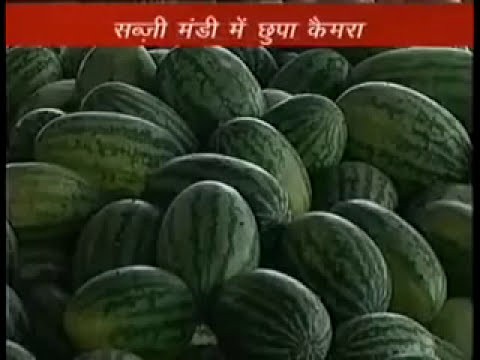The image depicts a multitude of watermelons in an outdoor market setting, characterized by its overall dark appearance. The watermelons, predominantly exhibiting a dark green hue with lighter green stripes, are piled haphazardly in various orientations. They vary in size and display an oval shape, with some showing yellow bruising, often indicative of their sweetness. At the top of the photo, a red bar spans across the frame, containing white text in a foreign script resembling Sanskrit or a similar language, though the exact meaning remains unclear. The lighting suggests a northeast directional sun, subtly illuminating the watermelons from the right side.